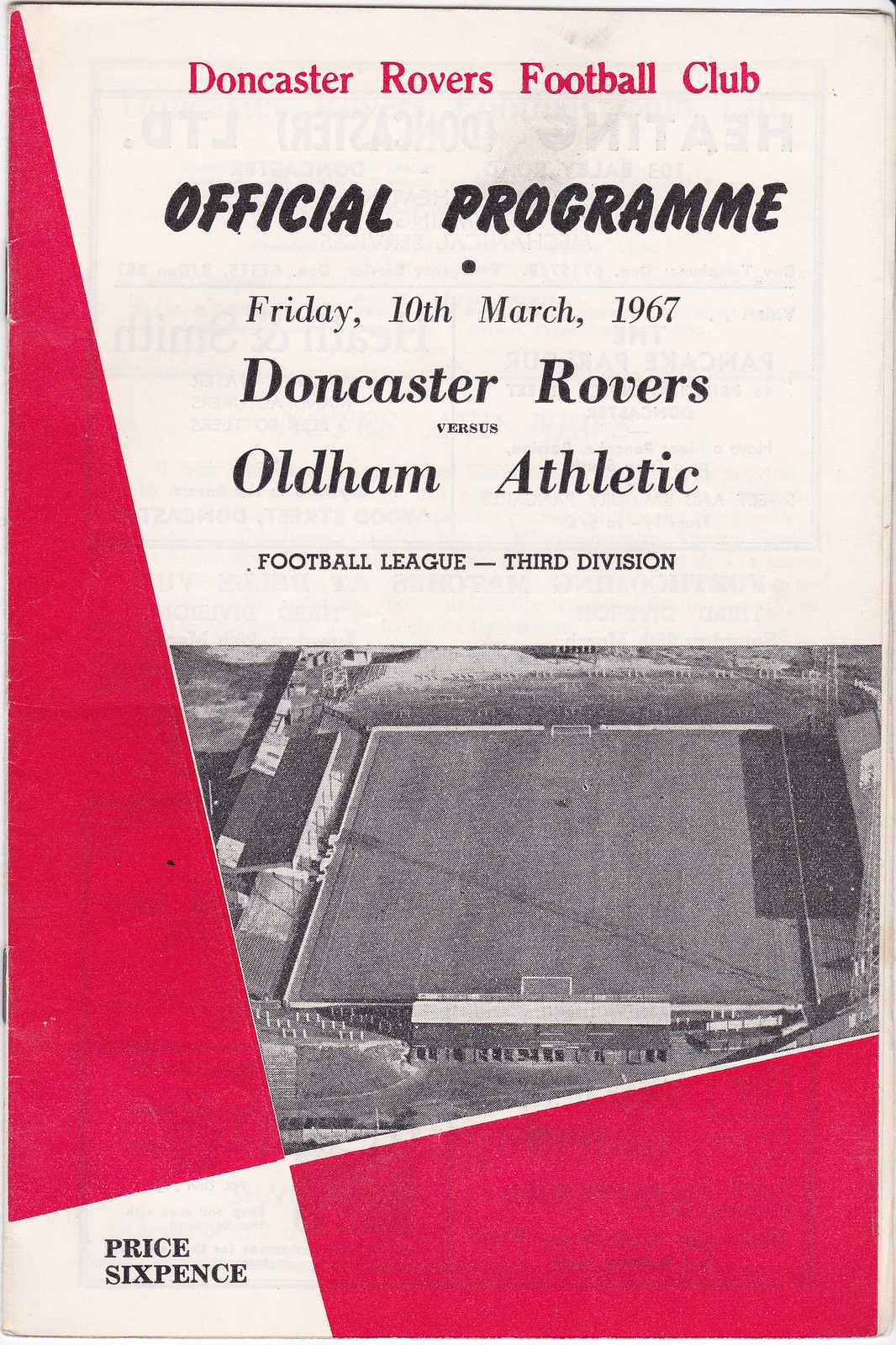This is an image of a vintage program from the Doncaster Rovers Football Club, dated Friday, 10th March 1967, for their match against Oldham Athletic in the Football League's Third Division. The program is visually striking with a combination of white and pink elements. Across the top, bold text reads "Doncaster Rovers Football Club Official Program." Beneath this, the date and match details, "Friday, 10th March 1967, Doncaster Rovers vs. Oldham Athletic, Football League 3rd Division," are clearly displayed. The lower portion of the program features a black-and-white sketch rendering an aerial view of their stadium, depicted with detailed outlines. On the left side, a large pink elongated triangle runs from the bottom toward the upper left corner, complemented by a smaller pink triangular square on the lower right corner of the image. Additionally, the price of "Sixpence" is noted within a white box located in the lower-left corner.